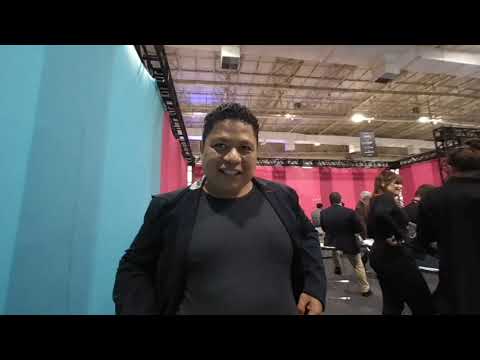The photograph is taken indoors, possibly within an exhibit hall or a large gymnasium-like space with an industrial, open ceiling. Central to the image is a medium-complected man with curly black hair, clad in a black t-shirt and a black collared jacket. He stands facing the camera with a partial smile. To his right, the camera-left, is a curtain wall adorned with vertical, two-toned light blue stripes, held up by black scaffolding. The background reveals curtains that transition into two shades of pink, also supported by black scaffolding. The floor appears to be either concrete or covered with a gray mat. Surrounding the man are six or seven individuals, all dressed in dark or gray tops, with one person wearing light tan khaki pants. None of the other people are looking at the camera, and they seem engaged in conversation or activities appropriate for a show or presentation. The overhead structure features visible metalwork and ductwork with ceiling lights that brightly illuminate the entire space. Main colors in the photo include shades of tan, black, blue, and pink.